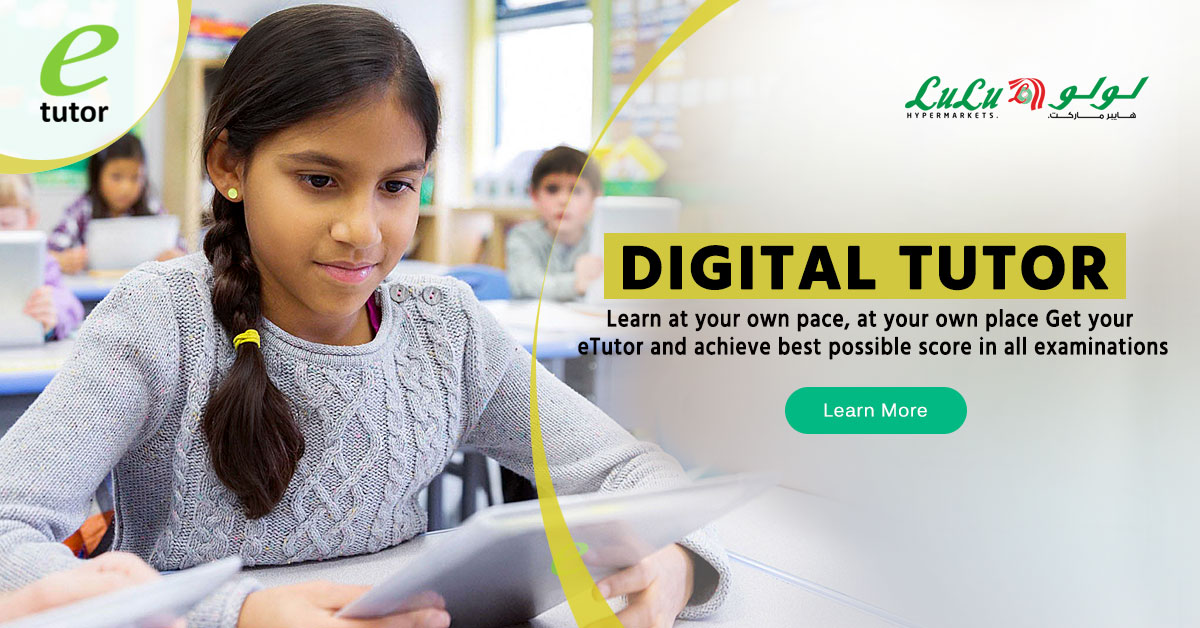The image is an advertisement showcasing E-Tutor. At the top left of the image, there's a logo for E-Tutor. The main photograph features a young Hispanic or Indian girl, approximately 10 to 12 years old, sitting at a desk in a classroom. She is wearing a gray sweater, has her hair in a braid and a ponytail, and is adorned with earrings. She is focused on a tablet in her hands. On her right, a little boy in a green shirt is looking directly at the camera. Over her left shoulder, there’s another girl of the same age, dressed in a plaid shirt, also engaged with a tablet.

The background reveals several other desks with students who are similarly occupied with their tablets. Additional elements in the background include walls with shelving and a window. 

On the top right corner, there is the logo for Lulu Hypermarkets. Adjacent to this logo, the text "Digital Tutor" appears in black on a yellow band, followed by the slogan "Learn at your own pace, at your own place. Get your E-Tutor and achieve the best possible score in all examinations." Beneath this, a green button reads "Learn more." The colors in the image include gray, white, green, red, yellow, black, purple, and blue, giving it a vibrant and engaging look. Overall, the advertisement emphasizes the convenience and effectiveness of the E-Tutor service in a learning environment.